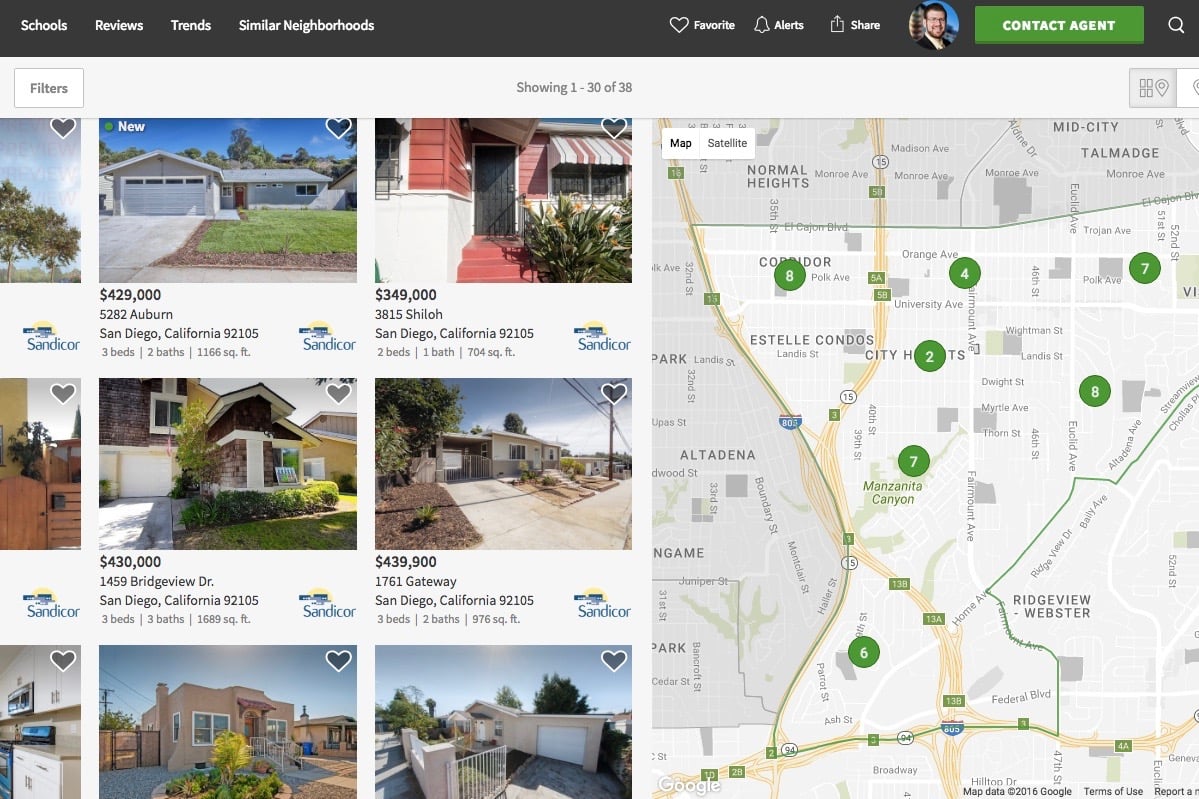This screenshot showcases a website dedicated to real estate in San Diego, California. The main focus is on the listing of homes for sale, ranging in price from $300,000 to $400,000. On the left side of the interface, there are six distinct images of large, attractive homes. Each of these homes is displayed with a thumbnail image that offers potential buyers a visual preview.

On the right side of the screen, there's an interactive map sprinkled with green circles, each containing numbers. These likely represent the locations of the available properties, along with major highways, freeways, and various city streets. This map provides an overview of the area and helps users understand the location of each listing in relation to key infrastructure and conveniences.

At the top right corner, there's a prominent green rectangular button labeled "Contact Agent," providing an easy call-to-action for interested buyers. The top left corner of the screen features navigational options including "Schools," "Reviews," "Trends," and "Similar Neighborhoods," allowing users to explore more detailed information and comparisons to assist in their home-buying decision.